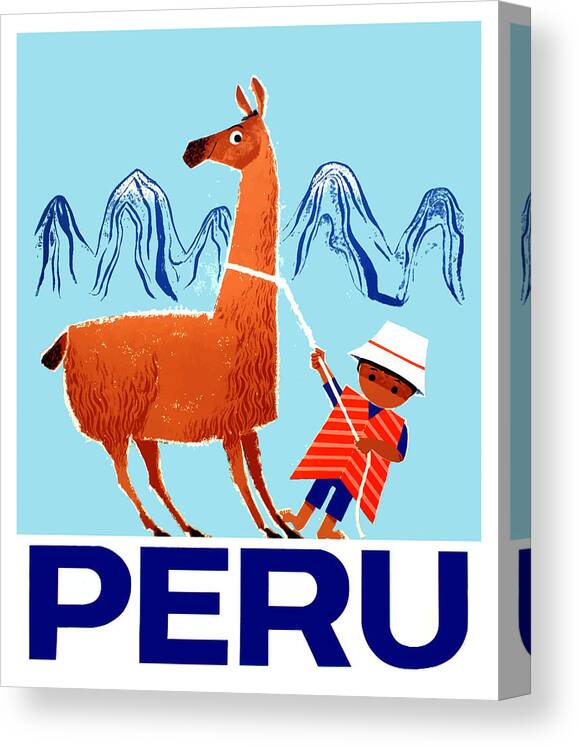The image depicts a vibrant, cartoon-like illustration set against a light blue background with wavy lines representing mountains. At the center, a boy with dark skin and dark hair, dressed in a red and orange striped vest over a blue shirt and blue pants, is shown leaning back while pulling a resistant brown llama with a white rope around its neck. The boy wears a white bucket hat with a red band and has a determined expression, though he lacks a mouth. The llama, looking backward over its left shoulder, contrasts with its tan fur and upright demeanor. In bold, dark blue letters at the bottom of the image, the word "Peru" is prominently displayed. The front of the box has a white border, and on the side, the same image is mirrored, with part of the "U" visible, suggesting a 3D or boxed canvas art piece.